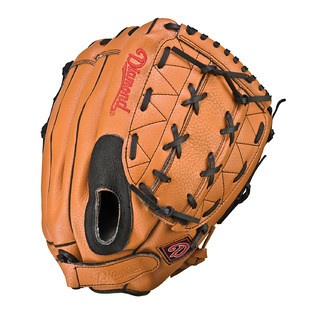This detailed photograph showcases a pristine baseball mitt, predominantly light brown or orangish-brown in color, set against a white background. The glove is shown from the back, revealing its intricate craftsmanship and fine condition without any scuff marks. It features black stitching running throughout, especially noticeable on the webbing and the edges. An X-pattern stitch is seen on the sides while the outer edge is secured with dark brown leather strapping.

Inlaid within the leather on the velcro strap at the bottom, as well as on the top half of the glove, appears the branding "diamond" in red cursive with an underline. Additionally, a black tag adorned with a red letter "D" on its inner side is located at the bottom right, reinforcing the brand's logo. The mitt includes a black-patched finger hole, designed for a right-handed thrower, indicating that the glove would be worn on the left hand.